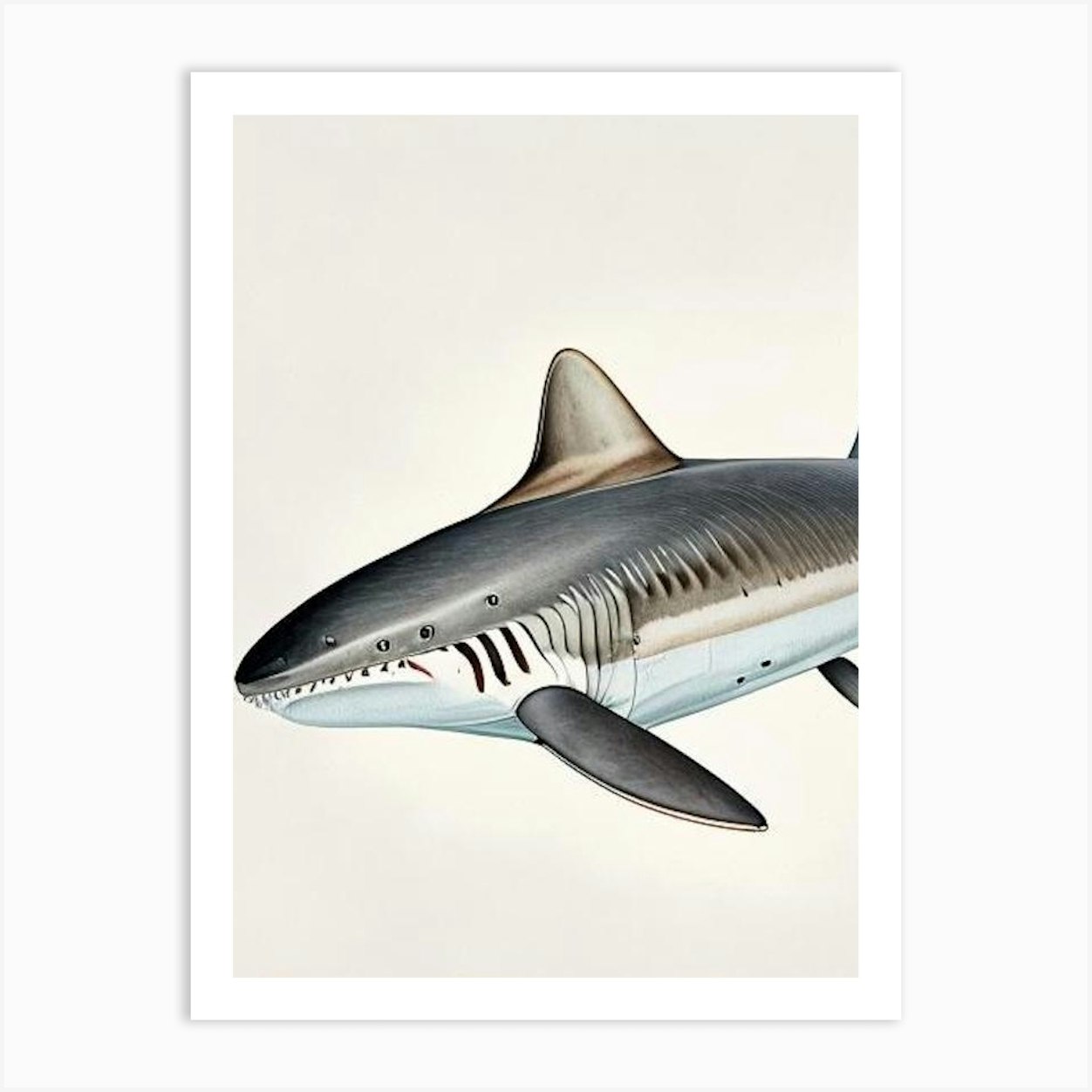This is an illustration of an unusual shark, set against a white or whitish-tan background with a light gray border. The shark itself closely resembles a great white shark in terms of shape but features unique and imaginative details that deviate from a real shark. Its body is predominantly dark gray to black on the top and white on the underbelly, somewhat reminiscent of an orca. There are numerous scales covering its body, and an odd metallic copper hue marks its dorsal fin, which contrasts with its pure black side fins. The shark's side features multiple eye holes rather than the expected single one, and its gills extend along the entire length of its left side, adding to its fantastical appearance. The shark's mouth reveals teeth that protrude slightly from its jaw. The drawing is presented on a piece of white paper, oriented vertically in a "hotdog" style frame. Notably, the image lacks any text or labels identifying this fictitious creature.